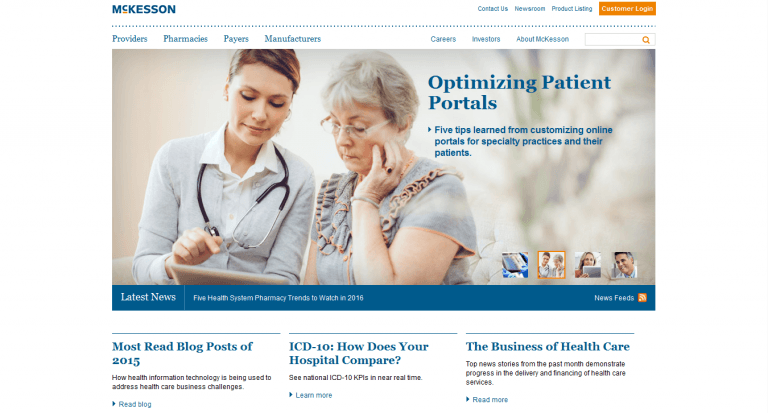The image is a detailed screenshot of a website in landscape orientation, likely displayed on a monitor or a laptop screen, belonging to McKesson. The McKesson logo sits prominently in the top left corner in blue, with the "C" distinctly smaller and raised. On the top right, an orange customer login button stands out. Next to it, there are blue links with the text "Contact Us," "Newsroom," and "Product Information," although the latter is partially obscured, possibly reading "Product Loading."

A blue dotted line spans across the screen below these elements, acting as a separator. Underneath this line, a navigation menu offers clickable links: "Providers," "Pharmacies," "Payers," and "Manufacturers" on the left; followed by "Careers," "Investors," "About McKesson," and a search bar with an orange magnifying glass icon on the right.

Dominating the webpage is a large photograph that covers approximately four-fifths of the screen, both horizontally and vertically. The image features an older woman with short hair and glasses, wearing a blue, ruffled shirt with short sleeves. She is holding her left hand up to her cheek and appears to be examining a clipboard or tablet held by a younger woman standing next to her. The younger woman, who has dark eyelashes possibly enhanced with mascara and her hair pulled up, is dressed in a white collared shirt, unbuttoned at the collar, layered under a gray sweater, and accessorized with a stethoscope around her neck, identifying her as a healthcare provider. She uses her right hand to point to or tap the tablet or clipboard.

Superimposed on the photograph is a blue bar with the text "Latest News," which is too tiny to read clearly. To the right of the older woman, text reads, "Optimizing Patient Portals: Five tips learned from customizing online portals for specialty practices and their patients," accompanied by an arrow indicating a link to this content. At the bottom right of the photograph, there are four thumbnail images, with the second thumbnail showing a smaller version of the main photograph of the two women, suggesting it is related to the article about optimizing patient portals. The content of the other thumbnails is unclear.

The bottom section of the screen is divided into three columns, each preceded by a very thin line. Each column heading is in bold blue font: the left column reads "Most Read Blog Posts of 2015," the middle column is titled "ICD-10: How Does Your Hospital Compare?" and the right column states "The Business of Health Care." Beneath each title is additional text and small, clickable "Learn More" or "Read More" expansion arrows.